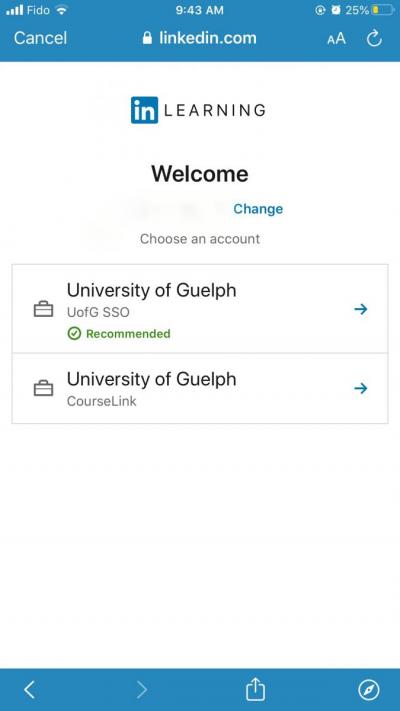The image shows a mobile device screen displaying a LinkedIn page. At the top, there is a blue horizontal bar, where in the upper left, the Wi-Fi network "Fido" is noted. Centrally, the time is displayed as 9:43 a.m., and directly below this, there is a padlock icon with "LinkedIn.com" written in white next to it.

In the main body of the page, set against a white background and positioned beneath the blue bar, is the word "Learning" with the LinkedIn logo to its left. Below this, the word "Welcome" is prominently featured in black text. To the right of "Welcome," in blue, it says "Change." Underneath this, in gray text, it reads "Choose an account." Two account options are presented below this instruction. The first option is labeled "University of Guelph, U of GSSO," with "Recommended" highlighted in green next to it.